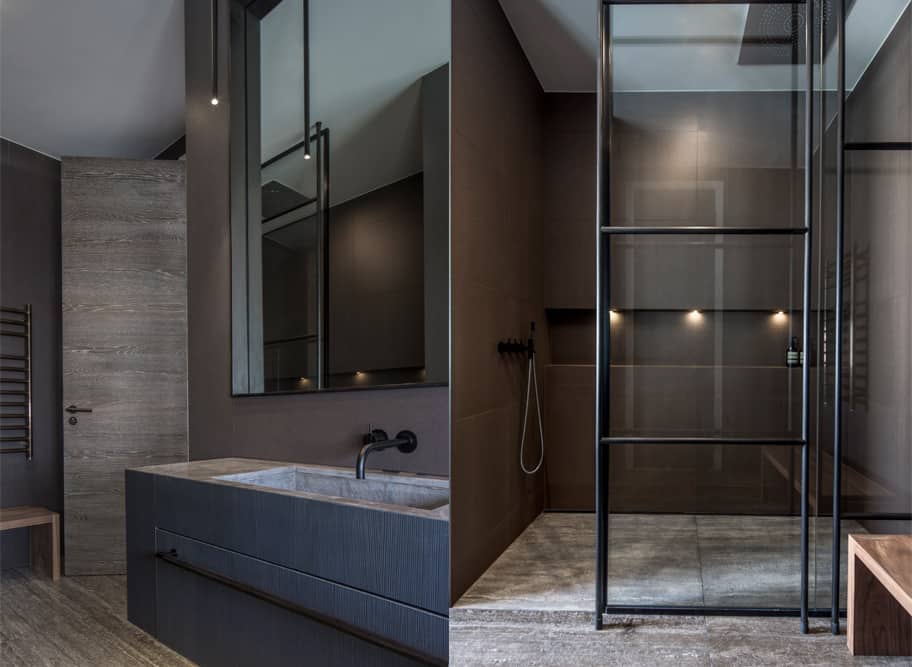This split image showcases two views of a highly modern, high-design bathroom characterized by a minimalistic, industrial aesthetic. The left side features a spacious gray stone sink set into a large, stone-looking base. A sleek, dark faucet complements the setup, positioned against brown-hued walls. Above the sink, an expansive mirror stretches nearly to the ceiling, flanked by two exceptionally thin, vertical tube lights, descending three to four feet from the ceiling, casting a contemporary glow over the space. In the background, there's a glimpse of a stool and possibly a piece of art, enhancing the room's sophisticated atmosphere.

The right side of the image presents a walk-in shower area with a striking glass door. This portion of the bathroom maintains the same avant-garde lighting scheme, although here the lights are arranged horizontally. The shower area emphasizes a seamless, uncluttered look, featuring a detachable showerhead and walls of dark stone or granite. A matching bench sits nearby, reinforcing the room's cohesive design with its modern yet functional elements. The overall color palette ranges from dark tan to different shades of gray, unified by granite and stone textures that highlight the bathroom's cutting-edge style.